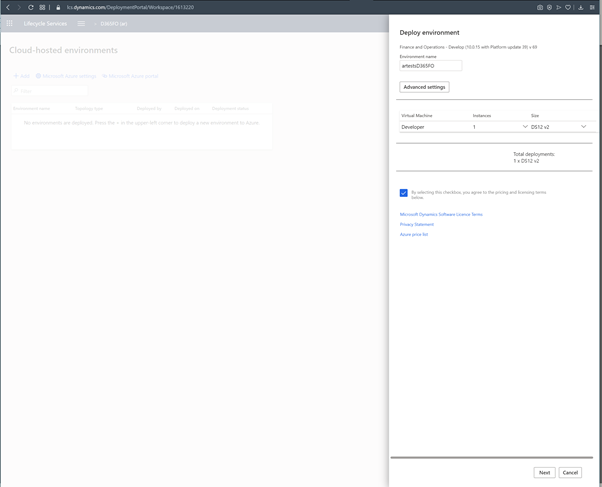The screenshot captures a detailed view of a web interface predominantly featuring the Microsoft Dynamics 365 Lifecycle Services (LCS) portal. At the very top of the image is a small web address reading "ks.dynamics.com" followed by an extensive query string. Below the address bar, on the left-hand side, a navigation panel prominently displays "Lifecycle Services."

Directly underneath this header, the section titled "Cloud-hosted Environments" is visible. Within this section, there is a dropdown menu followed by a segment containing various buttons with text labels, indicating different available functionalities.

On the right-hand side of the interface, a pop-up window titled "Deploy Environment" is prominently displayed. Directly beneath this heading, there is a smaller line of instructional text. A text box labeled "Environment Name" allows the user to input a specific name for the environment.

Below the text box, a button labeled "Advanced Settings" is available for further configuration options. The subsequent section titled "Virtual Machine Developer" lists two dropdown menus; the one in the middle has an unreadable label but displays the number "1," and the third dropdown menu has a label that reads "Size."

Towards the bottom of the pop-up, there is a checked checkbox with several links listed beneath it, likely offering additional options or information.